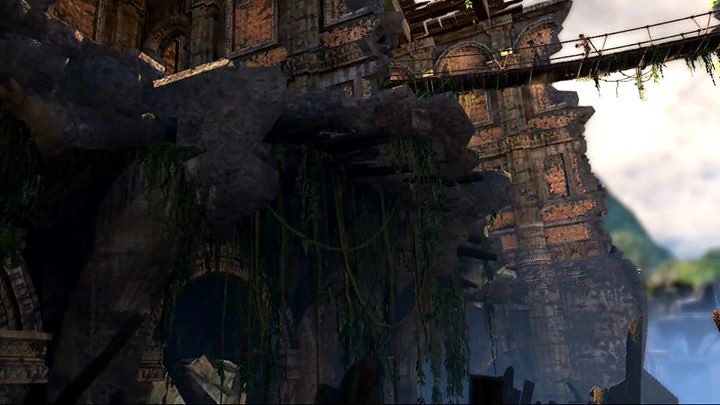This image, seemingly a still from a highly realistic video game, depicts a hauntingly beautiful, yet eerily desolate, historical scene. The focus is on an array of grandiose brown buildings, which, despite their ornate and towering structure, appear severely damaged. Their crumbling facades hint at a past cataclysm, whether through war, bombings, or simply due to the passage of time. Nature appears to be reclaiming its space; green moss and foliage hang down from the remnants of the structures, adding to the atmosphere of abandonment. Spanning between two buildings is a precarious, rickety bridge, adorned with strands of hanging moss, creating a foreboding pathway. Walking cautiously across the bridge is a lone human character, adding a sense of scale and narrative to the scene. In the backdrop, a verdant green hill rises, contrasting with the decaying architecture. Above, the sky is a pale, almost white, canvas dotted with ominous gray clouds, casting a muted light over the entire scene. The overall mood is one of melancholic beauty, blending decay with the persistence of nature.